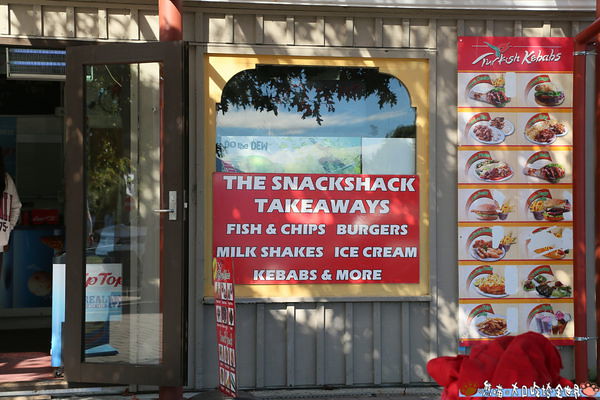The photograph depicts the exterior of a snack shop with tan to light gray wooden paneling resembling wainscoting. Central to the image is a window with a yellow frame, covered by a red sign displaying the text "Shake Shack" in white, advertising takeaways such as fish and chips, burgers, milkshakes, ice cream, kebabs, and more. To the right of this window, a tall sign prominently reads "Turkish Kebabs" at the top, and showcases around 14 colorful photos of various dishes arranged in two columns. On the left side of the window, there is a brown and glass door slightly ajar, revealing a glimpse of the interior where a half-visible person and a box can be seen, hinting at the shop's active environment.